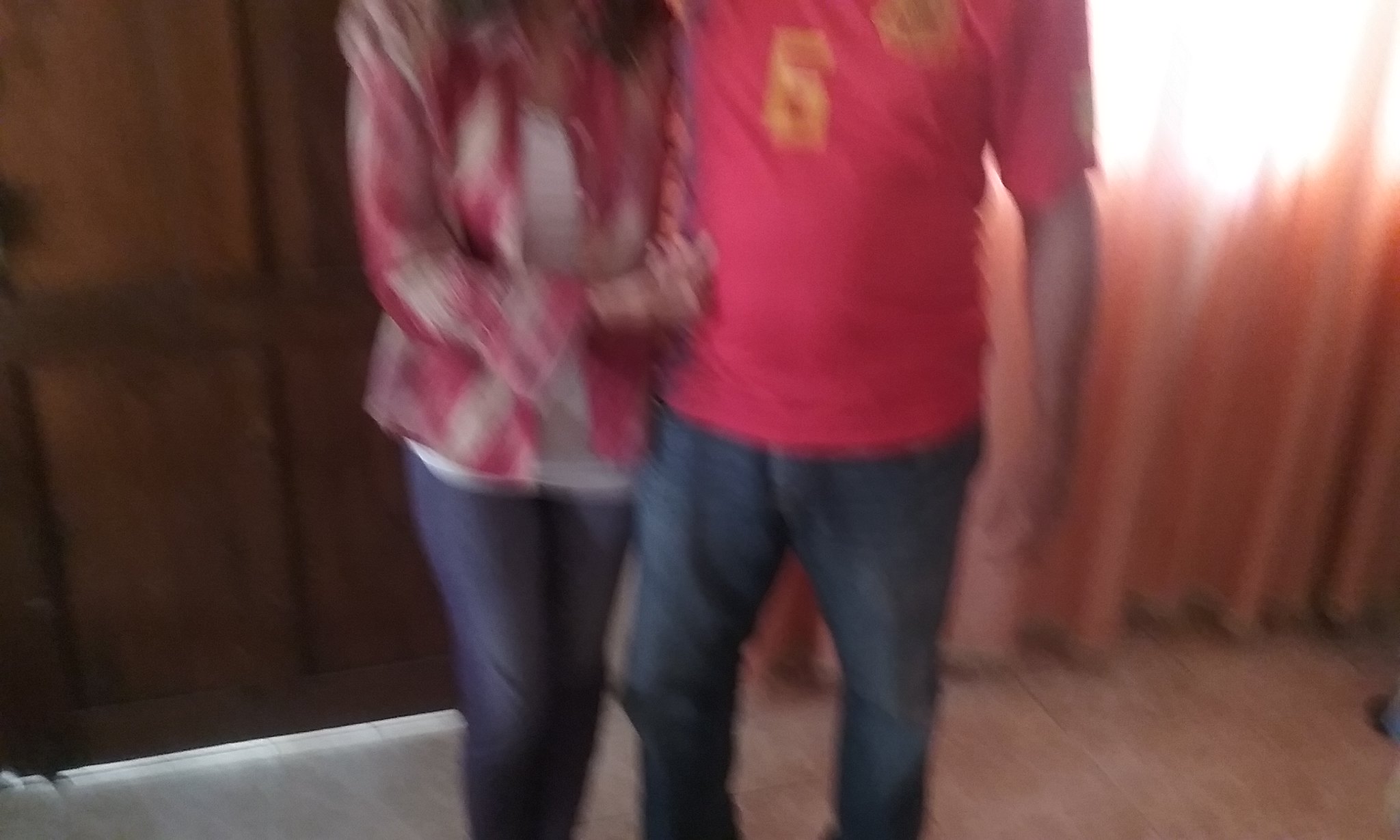This color photograph captures a casual moment between a couple from the shoulders down. The female figure stands on the left, closely positioned next to the male figure on the right. She clasps her hands in front of her, with her fingers near the man's midsection. Both individuals are dressed in relaxed, casual clothing. The woman wears a plaid shirt with shades of pink over a white undershirt, while the man sports a dark pink jersey-style shirt. They both pair their tops with jeans. The backdrop suggests a cozy home environment, accented by a curtain through which a bit of sunlight filters on the right side of the image. Although the photo is heavily blurred with no sharp details visible, it evokes the warmth and informality of a candid moment shared by the couple.